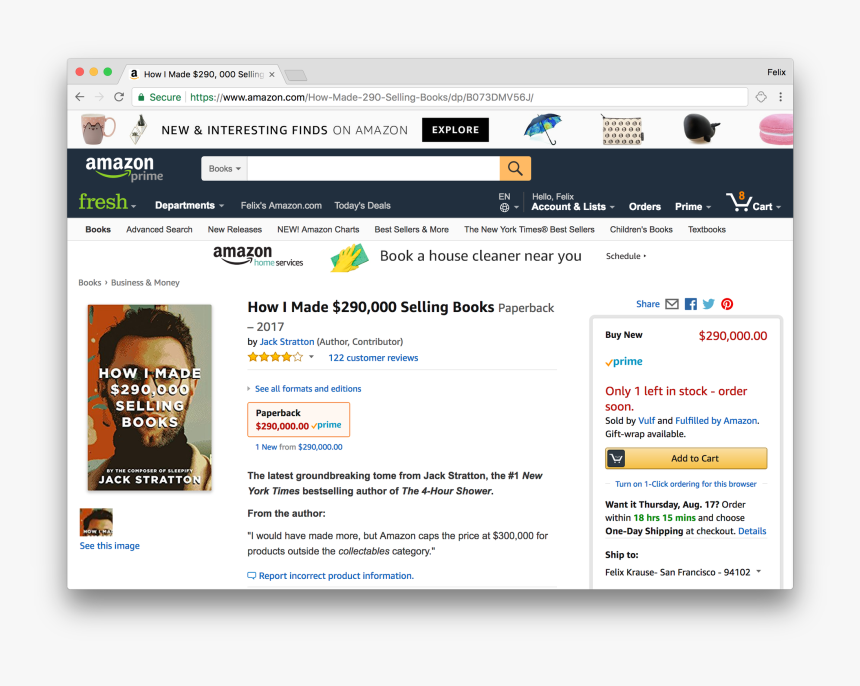In this image, we have a screenshot of an Amazon webpage open on what appears to be a Mac computer. The Mac interface is indicated by the typical red, orange, and green buttons in the top-left corner of the window. Moving right, we see the Amazon tab prominently displayed. In the upper right corner of the Amazon page, the name "Felix" is visible in black text, indicating the logged-in user. Below Felix's name, there is the combined search and address bar, followed by Amazon's signature blue banner that includes options such as "Amazon Prime" and "Amazon Fresh."

The blue navigation bar also features a search bar, as well as links to "Departments," "Today's Deals," "Hello, Felix," "Account & Lists," "Orders," "Prime," and a shopping cart icon that indicates there are eight items in the cart.

The focal point of the screenshot is a specific listing for a book titled "How I Made Two Hundred and Ninety Thousand Dollars Selling Books," authored by Jack Stratton. The book is priced astonishingly at $290,000, with only one copy left in stock. This item is available under the conditions of being "sold by both and fulfilled by Amazon."